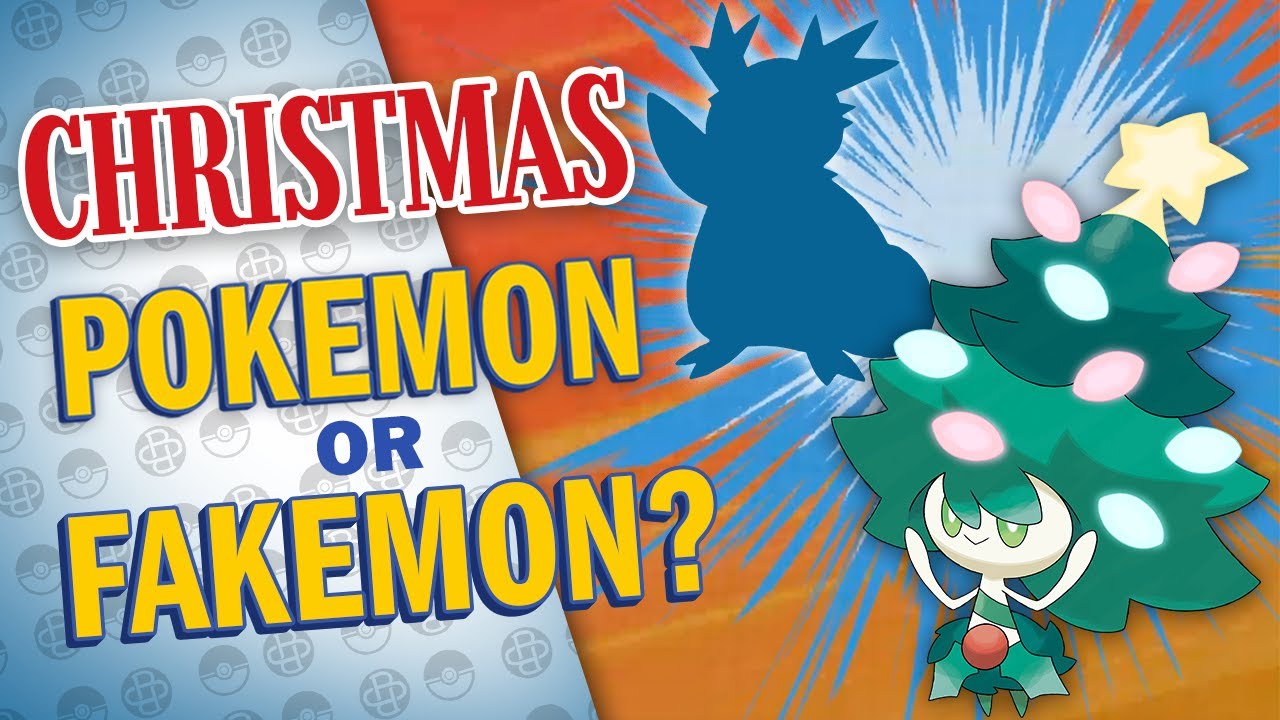This is a screenshot of a YouTube thumbnail designed in the style of Pokemon content, easily recognizable by its distinct art style and the word "Pokemon" prominently displayed. The thumbnail appears to advertise a Christmas-themed quiz or game, challenging viewers to determine whether certain designs are authentic Pokemon or made-up Fakemon.

On the left side of the thumbnail, the word "Christmas" is boldly written in festive red text with white highlights, creating a holiday ambiance. Just below it, the words "Pokemon or Fakemon" are featured, hinting at the nature of the game or quiz.

To the right, the image showcases two different Pokemon designs. The upper-left corner features Delibird, often associated with Christmas due to its penguin-like appearance and Santa Claus-inspired red and white color scheme, complete with a sack. In the bottom-right corner, there is a whimsical Fakemon characterized by a Christmas tree on its head, adorned with red and blue lights and topped with a star. This creature has green eyes and appears to be holding the tree with its hands.

The overall layout and festive elements of the thumbnail effectively communicate the holiday theme and the interactive nature of the content, inviting viewers to engage in a fun and seasonal guessing game.